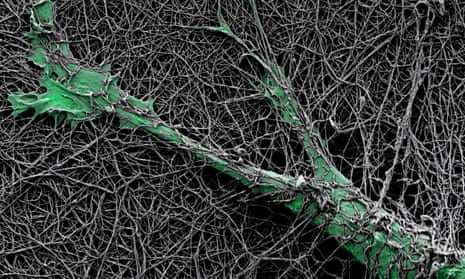The image portrays an intricate and dense web of thin, dead branches sprawled chaotically across a flat surface, reminiscent of a tangled root system. Intertwined among these branches is a vivid green vine that diagonally stretches from the bottom right to the top left. This vine features a distinct V-shaped structure with two branches extending outward, possibly terminating in leaf formations. The dead branches appear to wrap around and support the green vine, creating a complex and dynamic scene. In the background, certain darkened areas suggest depth and incomplete coverage, creating a striking contrast against the densely woven, almost nest-like arrangement of the branches. This dense network, evocative of plant roots or swamp vegetation, brings to mind a naturally crafted formation that could be found in a wetland habitat. The image’s detailed and magnified perspective provides an almost microscopic view, emphasizing the textural and structural complexity of this natural phenomenon.